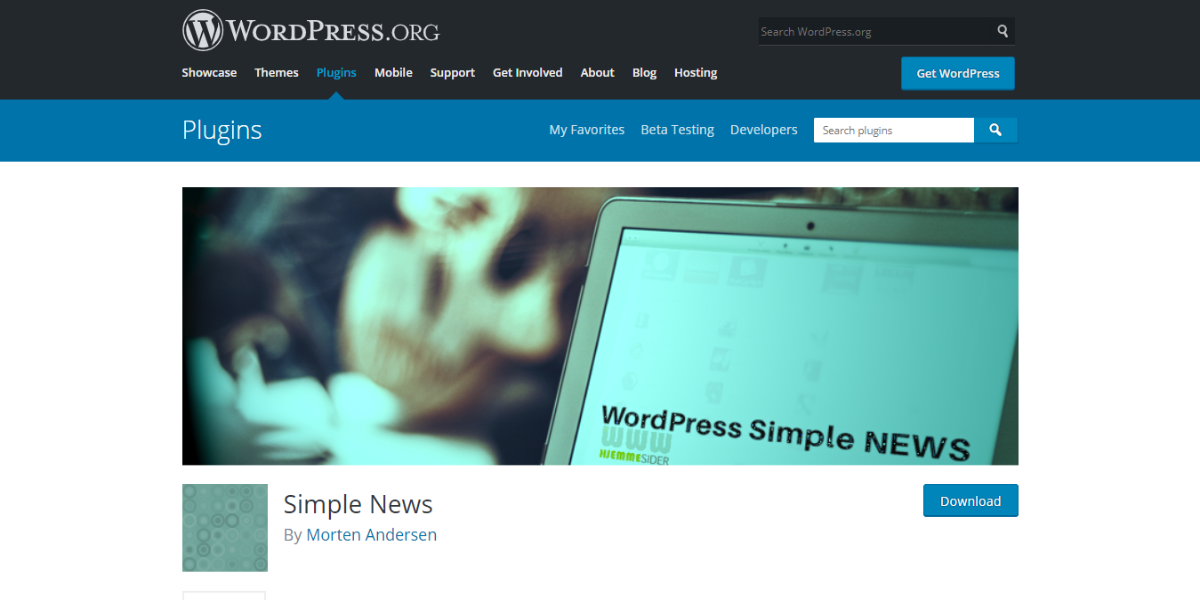The image shows the WordPress.org website interface. At the top, there is a black banner displaying the WordPress.org logo. Directly underneath this banner, a navigation menu offers several options: Showcase, Themes, Plugins, Mobile, Support, Get Involved, About, Blog, and Hosting. To the right of the navigation menu, there is a 'Get WordPress' button and a magnifying glass icon for search functionality.

The screen view indicates that the user has clicked on the 'Plugins' option from the menu. This action activates a blue bar directly below the black banner, now highlighting the 'Plugins' section. This blue bar includes further options: My Favorites, Data, Testing, Developers, and a search bar accompanied by another magnifying glass icon for plugin-specific searches.

Below this, the main content of the page displays a featured plugin. The plugin is presented in a rectangular image with a blurred background, showcasing an open laptop. On the laptop's screen, the text "WordPress Simple News" appears prominently, along with the stylized WordPress "W" logo. Below the logo, it says "Simple News by Morton Anderson." There is also a 'Download' button available for users who wish to obtain this plugin.